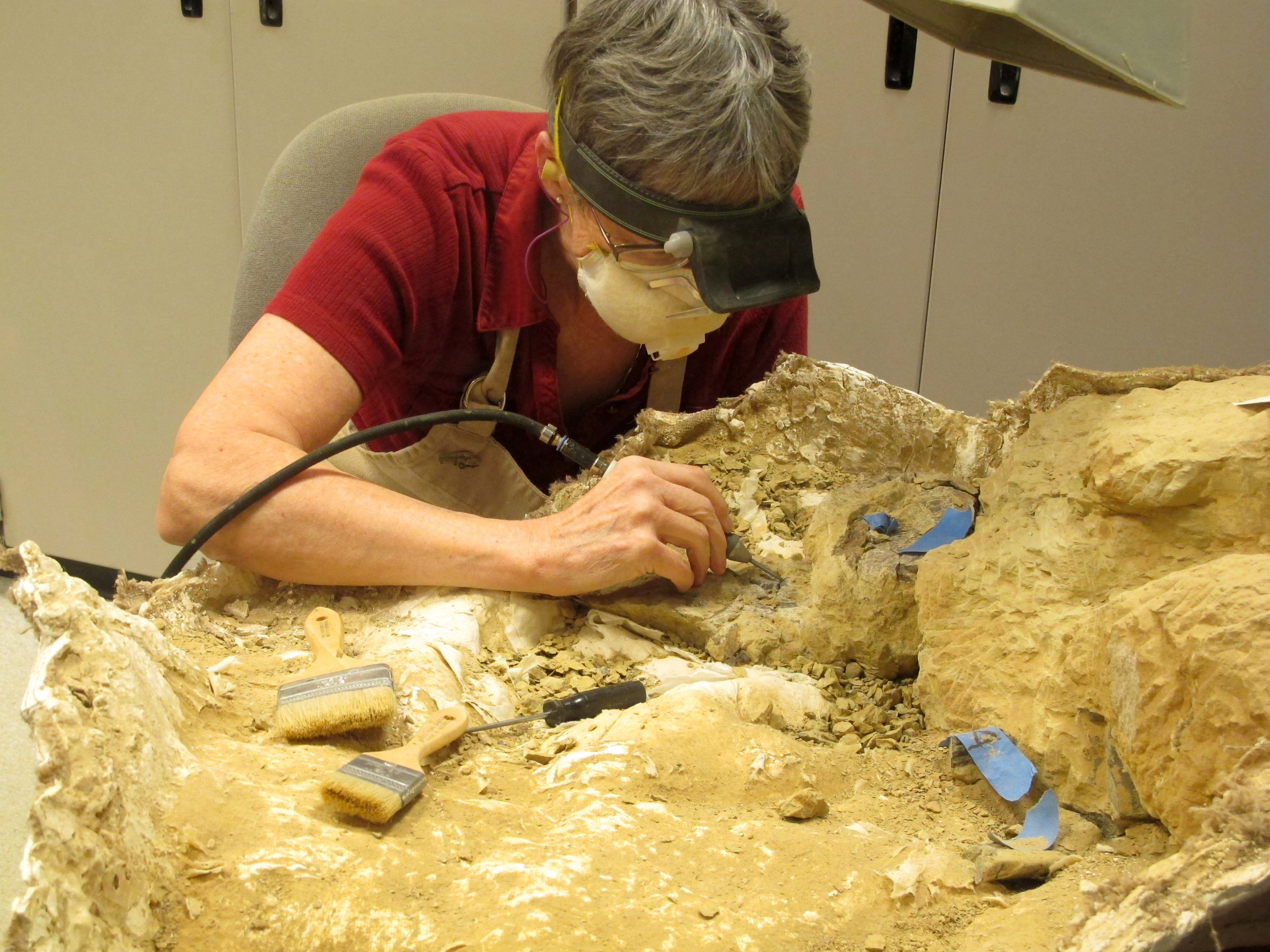A rectangular image depicts an older woman, likely a professional archaeologist in her 60s or 70s, meticulously working on a large rock formation in an indoor setting. She has short gray hair, wears glasses, and is outfitted with a white face mask and a small headlight headband for better visibility. Her attire includes a red short-sleeved polo shirt. She sits in a gray office chair, intently focused on chiseling the rock formation with a pen-sized agitator connected by a black cord. Surrounding her on the table and nearby shelving are various brushes and small black-handled tools. Red painter’s tape marks specific areas on the rock, which has striking blue chunks embedded in it, hinting at valuable archaeological or organic material. The detailed backdrop, including a white wall with shelving, emphasizes the controlled and methodical environment of her workspace.